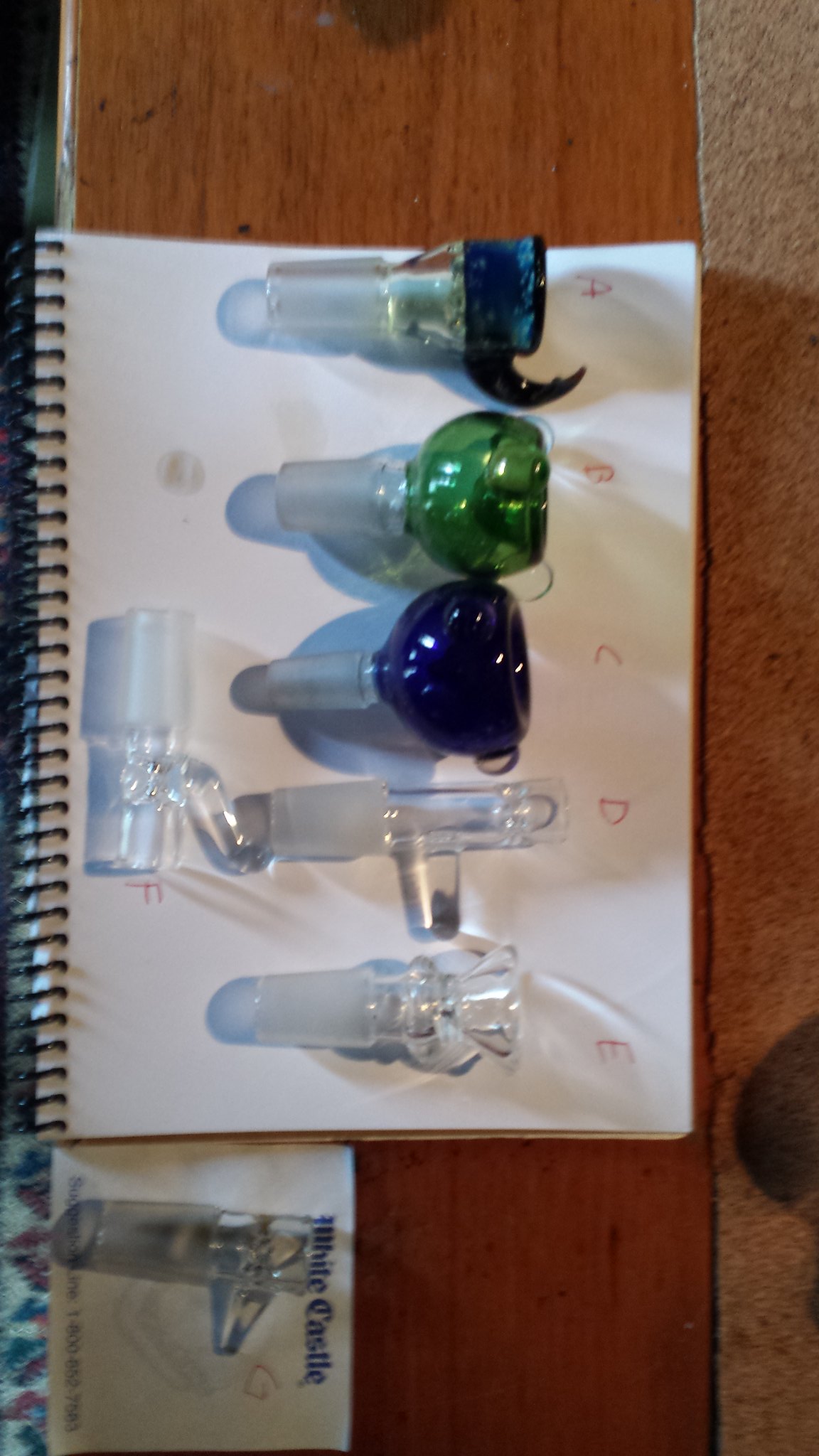The color photograph depicts a collection of smoking paraphernalia, traditionally used for inhaling narcotics such as cannabis. The image has been rotated 90 degrees anticlockwise, and for accurate description, it should be visualized in its correct orientation by turning one's head 90 degrees clockwise. The paraphernalia, often resembling hookah pipes or bowls for tobacco, rest on a white piece of paper attached to a spiral-bound notebook. The notebook lies on a reddish wooden surface, possibly a table or floor.

On the piece of paper, each item is labeled with a letter, from A to E sequentially from left to right, with an additional letter F noted on the left side of the page. Above each item, the respective letter is inscribed in red pen. Bombs A, B, and C appear inverted, with their inhaling tubes pointing downward and their conical bases upwards. Each piece is unique in shape and size, with A and C showcasing blue glass bottoms—C being the darker shade—and B displaying a green glass base. The arrangement hints at this being categorized or examined evidence, possibly from a crime scene, given the meticulous labeling and documentation.